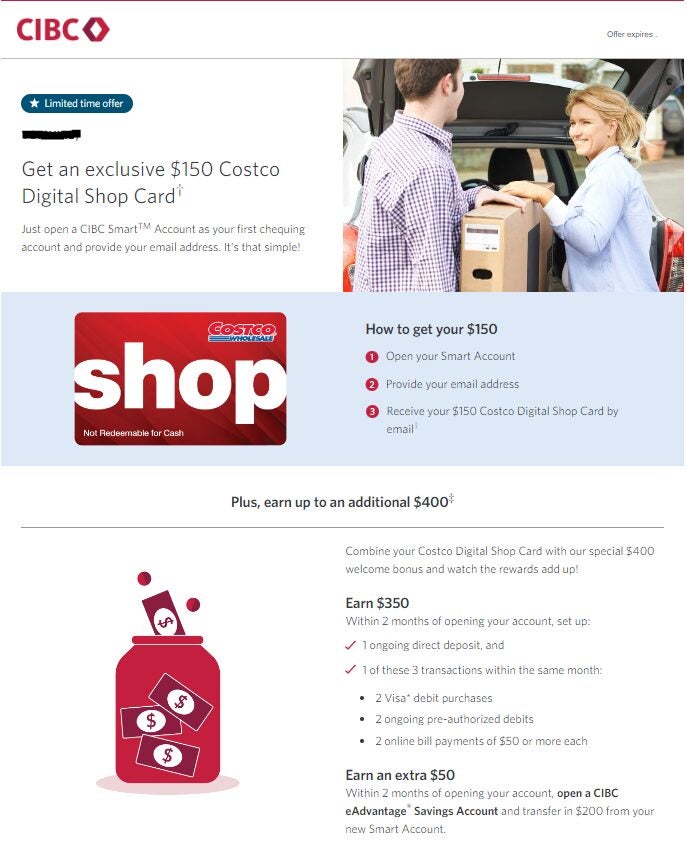This image is a promotional screenshot featuring an advertisement for a Costco-related offer from CIBC. At the top, a thin red line divides the header from the content below. In a white space with all capital letters, "CIBC" is prominently displayed, accompanied by a hollow diamond symbol to its right. To the far right, the text "Offer Expires" is clearly visible, separated by a gray line beneath it.

Below this section, a distinctive blue-turquoise button with a white star icon is highlighted. The button's text, in white, reads "Limited Time Offer." Across a small, horizontal black bar beneath the button, the offer is introduced with the text: "Get an explosive $150 from Costco Digital Card." 

Further details instructing how to obtain this reward are included, starting with an invitation to open a CIBC smart account. Following this, a blue box with text minimally highlighting "Costco Card Shop – Not redeemable for cash" is shown. Clear steps labeled "1, 2, 3" in three circles detail the process for claiming the offer.

Additional promotional content reveals the potential to earn an extra $400, with instructions provided below. The imagery includes a red jar with money symbolizing potential earnings.

The advertisement is densely packed with visually distinct sections and instructional elements, all focused on highlighting the lucrative offer to attract customers to open a CIBC smart account and engage with Costco for financial rewards.